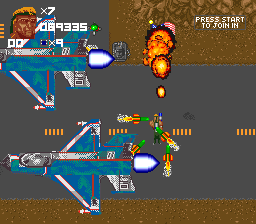This image appears to be a squared screenshot from a video game, depicting a dynamic and action-packed scene. Dominating the top right corner, the text "Press Start to Join" is prominently displayed in white font. Just below, there is a character's face featuring yellow hair and muscular features, accompanied by the number "9335."

In the main focus of the image, there are two blue planes both situated on gray runways lined with orange stripes. These planes, which resemble fighter jets, are positioned to the left, each exuding bright bluish-white flames from their engines, suggesting they are ready for takeoff or in mid-action. One of the planes at the top left appears mid-flight or has just taken off, while the lower plane is on the runway, preparing to follow suit. The lower portion of the image has a brown, dirt-like border, adding to the gritty atmosphere of the airbase.

Further adding to the chaos, there's an explosion close to the center-right of the image, with a large fireball breaking apart into smaller pieces of fire. Behind the lower plane, there seem to be some people and possibly additional aircraft. Additional details include elements like rockets or bombs emerging from one of the planes, emitting flames, and what appears to be a character wielding a green gun near the middle.